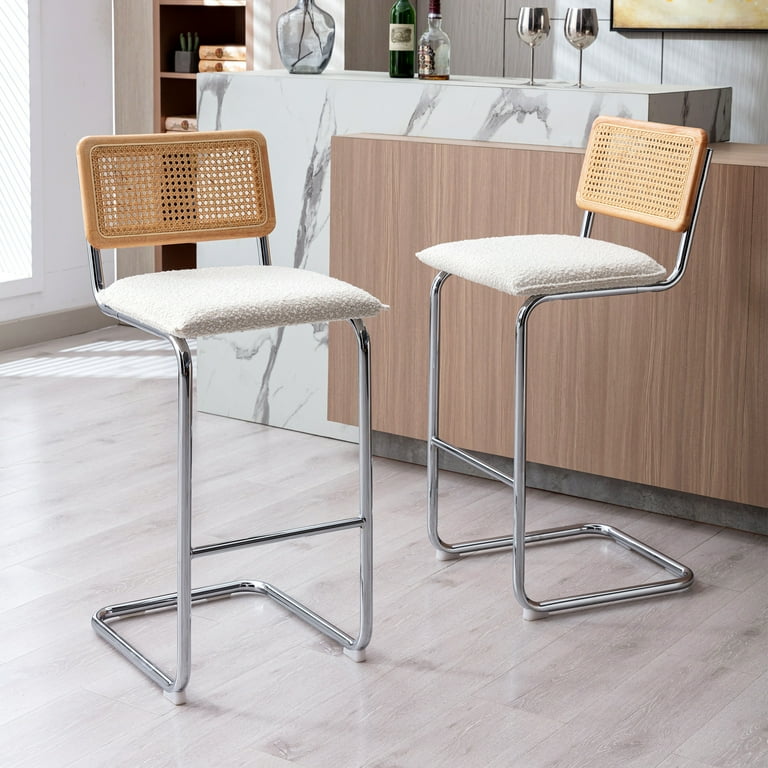The photograph, clearly staged and taken indoors during the daytime, captures a stylish corner of someone's home bar area. The image, vertically rectangular without a border, showcases a bright and inviting setting. In the upper left corner, a white door with a full window allows sunlight to pour into the room, casting a warm glow. Prominent in the background is a counter divided into two distinct sections: a white marble countertop and an adjacent wooden one. The marble section hosts two elegant wine glasses, a near-empty clear alcohol bottle, a green liquor bottle with a white label, and a clear glass vase holding some sticks or stems. Below the counter, the floor appears to be wooden or imitation wood. Dominating the foreground are two stool-height chairs with polished silver metal frames. Each chair features a cushioned white seat and a wicker backrest. The unique design of the chairs, with legs that extend down from the front before angling out into an L shape for support, adds to the modern aesthetic of the space.